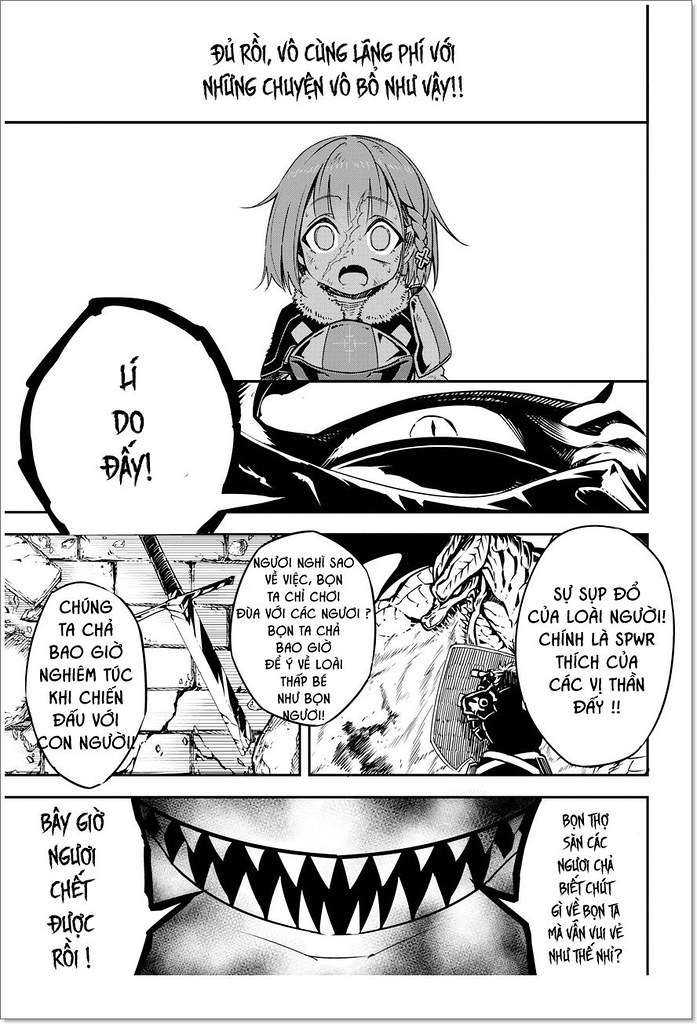This is a scanned black-and-white image of a page from a manga-style anime comic, likely in Vietnamese. At the top center, the text reads "Du Roy Vu Bo Kong Lang Phi Boi Nung Xuan Bao Bo Nu Ve!!". Below this, the next panel depicts a young girl with wide, frightened eyes and her mouth agape, accompanied by the words "e do day". The following panel zooms in on what appears to be a monster’s eye. Beneath this are three chat bubbles with text: "Chung Te Chau Bao Goi Ning Tuck Kee Chin Dao Voi Kong Nua", and to the far right, "Su Sep Do Ku Loi Nung Chin La Spur Dek Kao Kak Ve Thanh Day", though one bubble is too blurry to decipher. The final panel shows a close-up of a menacing, jagged-toothed mouth with the text "Bay Giao Nang Chet Juk Roi" on the left, while the right side remains illegible due to blurriness. To the upper right of the page, there seems to be an image that might resemble an evil eye, and possibly a dragon.